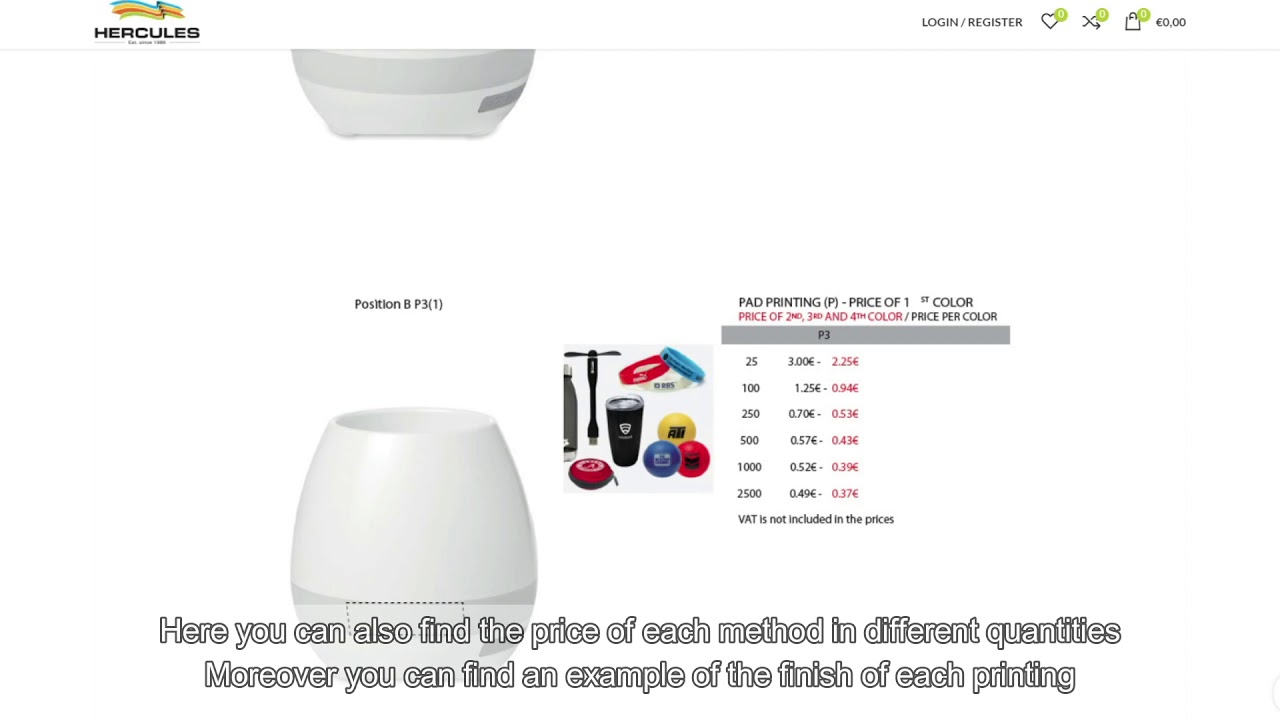The screenshot appears to be from a website named "Hercules," which is prominently displayed in the upper-left corner, accompanied by a colorful banner in blue, yellow, and red. To the right of the header, there are options for login and registration, along with icons representing a heart, an "X," and a shopping bag.

The page has a predominantly white background. At the very top left, part of what seems to be a white container is visible, followed by an area of white space. Below that, there's an image of what might be the same white container, resembling a diffuser.

Adjacent to the container image, a small picture features various pieces of sports equipment: a black cup, a red and blue ring, and several balls in blue, yellow, and red.

To the right of this image, text reads: "Pad Printing." This section outlines the pricing structure: the cost for one color, and additional costs for a second, third, and fourth color. Below, a detailed chart presents numbers alongside their corresponding prices.

At the bottom, a note states that users can find the price for each method in different quantities. Additionally, the page showcases examples of the finish for each printing method.